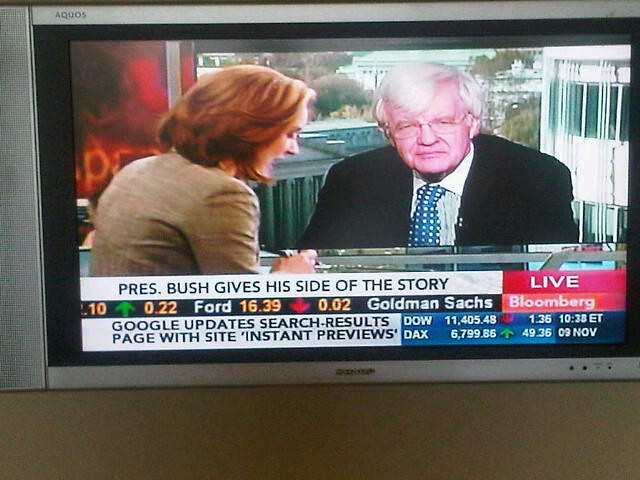The image captures a photograph of a TV screen showing a live Bloomberg TV news broadcast dated November 9th at 10:38 Eastern Time. The broadcast features a woman interviewer with short red hair and a business outfit, standing on the left side, seemingly reading into a microphone. On the right, there's a screen displaying a man with grey hair, glasses, a black suit, and a blue tie. The onscreen text reads "President Bush gives his side of the story," indicating the topic of discussion. Below this, a news ticker provides financial updates: Ford and the Dow are down, while the DAX is up. Additionally, it mentions that Google is updating its search results page with site instant previews. The broadcast is marked as live with a red and orange box in the bottom right corner.